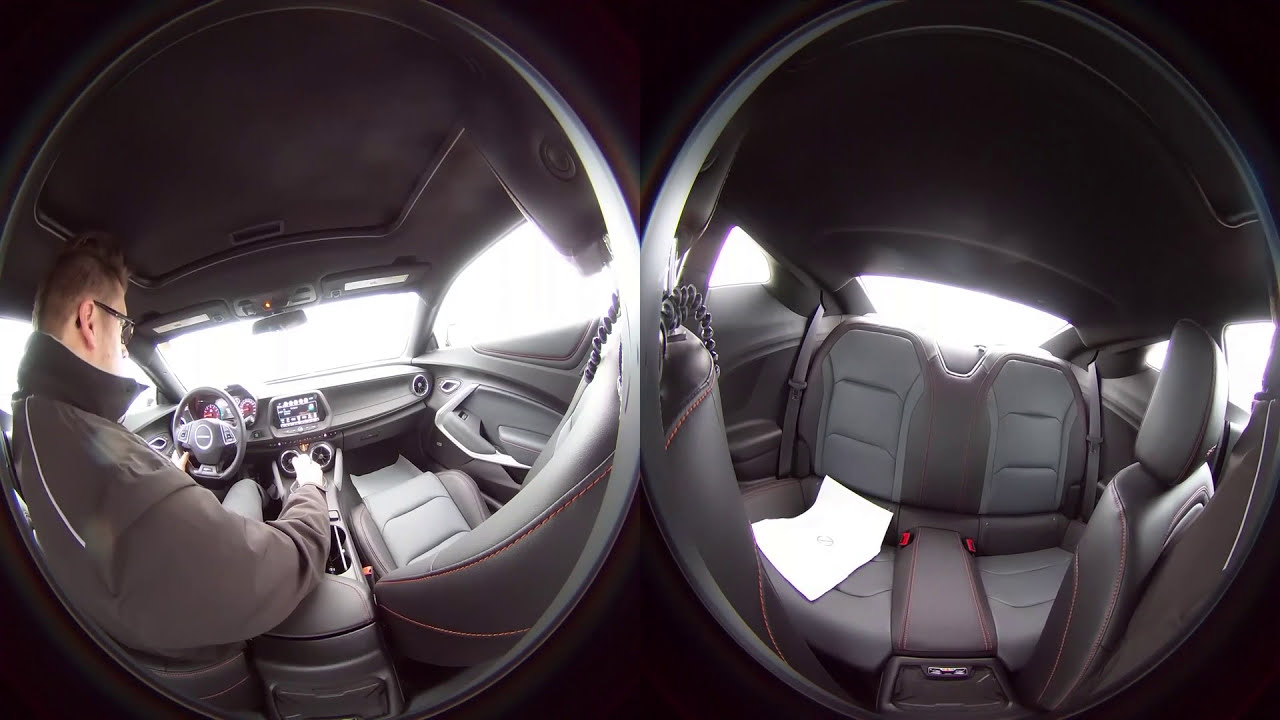This photograph captures the interior of a vehicle through two circular fisheye lens views. The left-side image, taken from the back of the car, shows the driver with one hand on the steering wheel and the other on the gear shift. This view also includes the driver's seat, the front passenger seat, and the front windshield, through which bright daylight streams in. The right-side image, captured from the front windshield, focuses on the two back seats. The back seats are empty except for a single white sheet of paper on one of them. The interior seats are a combination of gray and brown hues. Additionally, the vehicle features a sunroof, highlighting the daytime setting. Together, these images offer a comprehensive view of the vehicle's cabin, emphasizing its emptiness except for the driver.